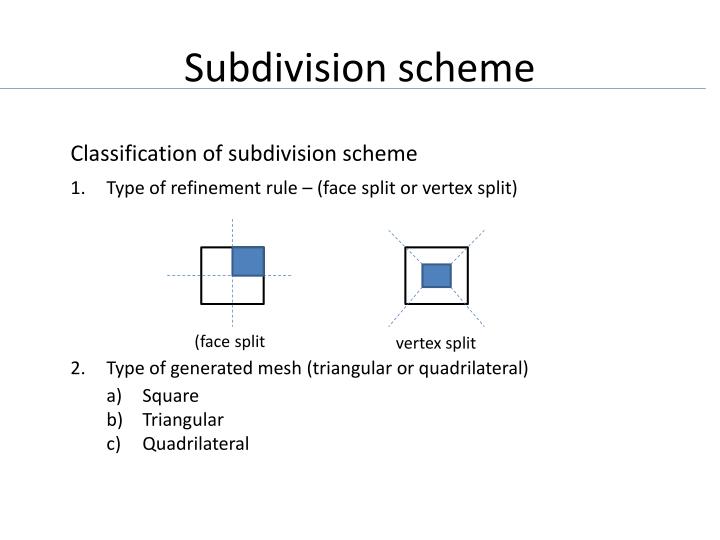In this presentation slide titled "Subdivision Scheme" at the top, separated by a horizontal blue line, the content is a detailed explanation of the classification of subdivision schemes. The first section, labeled "1. Type of Refinement Rule," describes two types: "Face Split" and "Vertex Split." Below this are two images depicting these rules. In the first image, labeled "Face Split," a large square features a smaller blue square in the upper right corner with a dashed cross slicing through the main square. The second image, labeled "Vertex Split," shows a smaller blue square centered within the larger square, also marked by a dashed cross. Following this is the second section, labeled "2. Type of Generated Mesh," which outlines that the mesh can be either triangular or quadrilateral. Subsections "a," "b," and "c" further break this down into Square, Triangular, and Quadrilateral meshes, respectively. The slide uses a clean white background with black, blue, and possibly gray elements, arranged in a structured, easy-to-read format reminiscent of a professional PowerPoint presentation.